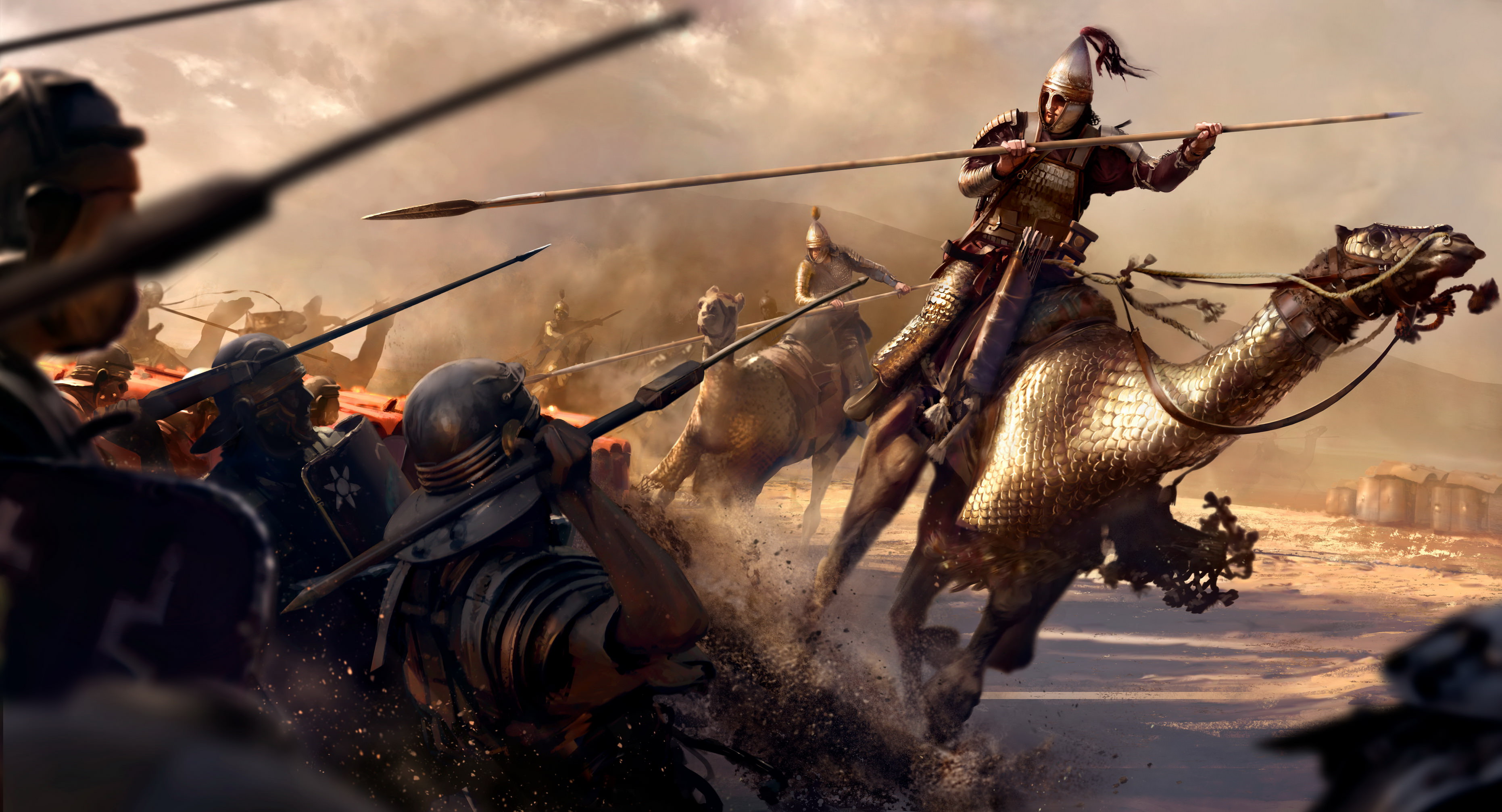This highly detailed 3D digital illustration or possibly a cutscene from a video game portrays an intense battle scene set in an alternate reality. On the right side of the image, heavily armored men ride on equally armored camels, their metal helmets adorned with pointy tops and tassels. These warriors brandish long spears and appear to be charging aggressively towards their opponents. The camels themselves are covered in protective metal armor on their heads, necks, and flanks, matching the metallic and leather armor of their riders.

On the left side, a group of men on foot brace themselves at the edge of a sandbar, preparing for the imminent attack. These ground fighters are also clad in heavy armor, with round helmets featuring wide brims to protect their necks. Many of them hold shields in a desperate attempt to defend against the incoming assault, while others are poised to throw their own spears towards the mounted attackers. The scene is set under a dramatic sky, with storm clouds gathering on the left side, juxtaposed against rays of sunlight breaking through and illuminating both the foot soldiers and the camel riders. In the background, on the right side, the faint outline of a city can be seen, adding to the historical or fantastical backdrop of the sandy battlefield.